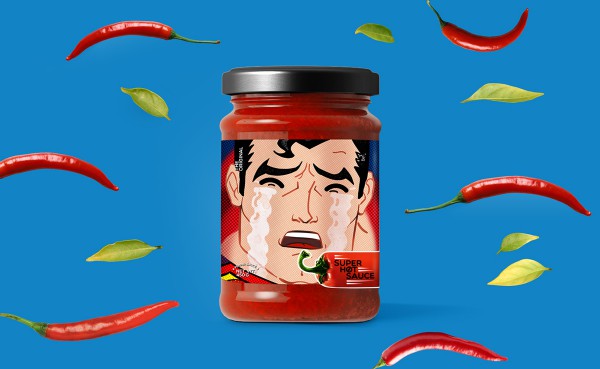The image is an advertisement featuring a mason jar filled with red chili paste, prominently displayed against a blue background. This mason jar, topped with a gray lid, bears a distinctive label. The label showcases a cartoonish, muscular Caucasian man, resembling the comic book version of Superman, complete with his sharp eyebrows and iconic tuft of hair. The man's expression conveys extreme discomfort; his mouth is open, revealing the top row of white teeth, and large tears stream down his face. This dramatic depiction suggests the intense heat of the product inside the jar. Surrounding the jar, there are red long hot peppers and green leaves, with an arrangement of six peppers and six leaves floating around it. The label also features a drawing of a red hot pepper with a green stem. At the bottom right corner of the label, the text within the pepper reads "Super Hot Sauce," emphasizing the product's fiery nature.